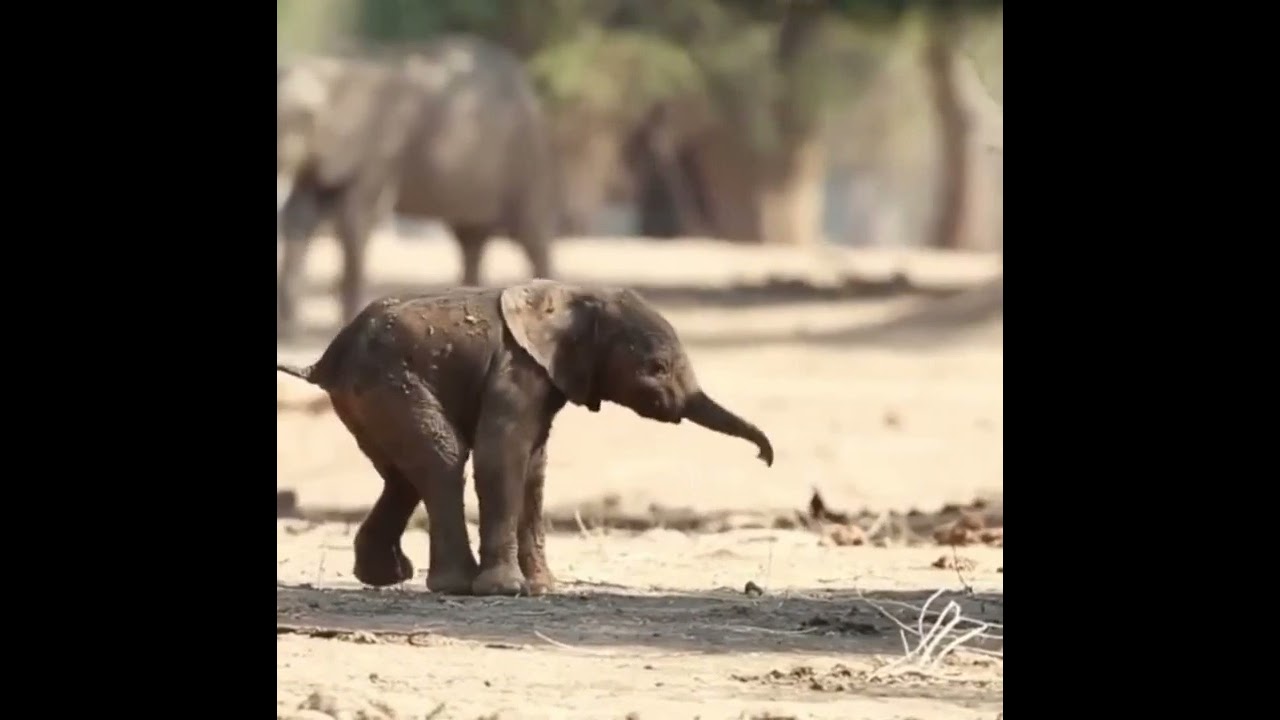In this detailed photograph, we see an adorable baby elephant in the foreground, facing to the right. His back left leg is lifted slightly off the ground, while his other three legs are firmly planted. His trunk curves downwards, and his tail is straight out behind him, although partially out of the frame. His ears are flattened against his body, and he has an open eye, appearing alert and curious about his surroundings. 

The baby elephant stands on a dirt surface strewn with leaves, twigs, and rocks, some of which are visible on his back. He is partially in the shade, with some areas illuminated by sunlight, enhancing the texture of his tannish-brown skin and hinting at slight motion, as if he is walking or about to take the next step.

In the background, a larger adult elephant, possibly his mother, stands slightly to the side. This adult elephant, along with a backdrop of trees with leaves, is blurry, suggesting the use of portrait mode to emphasize the sharp clarity of the baby elephant. Overall, the photograph beautifully captures the essence of the young elephant's curious and lively nature.